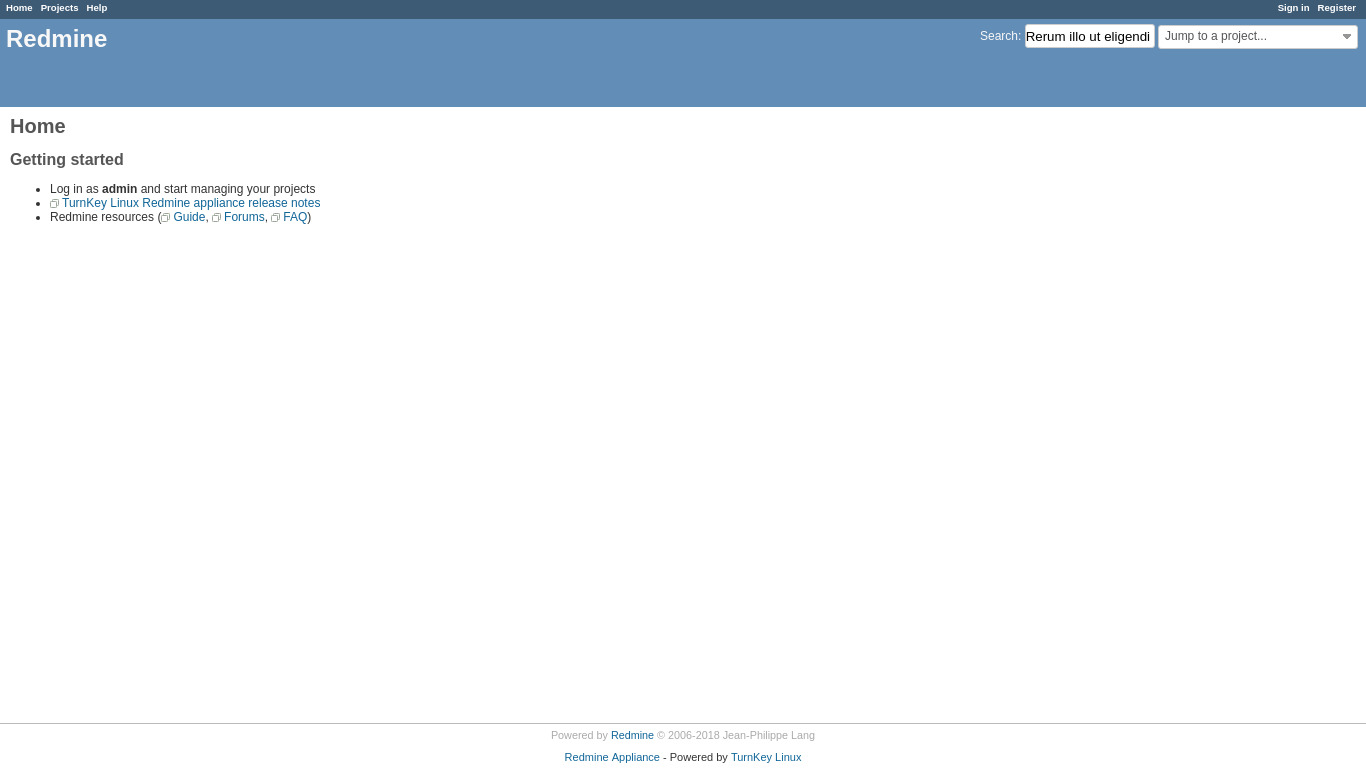**Detailed Caption:**

The image features a two-tone blue interface with white text predominantly used for headings and labels. At the top, in a blue header with white font, the text reads "Home Projects Help," and towards the right, the words "Sign-In Register" are visible.

Directly below this header, a slightly different shade of blue serves as the background for the label "RedMine." The label is styled as a single word with each letter capitalized in white: "REDMINE". Adjacent to this, a search bar is displayed with the placeholder text "Search..." inside a white rectangle. Below this, there is a line of text in black, written in a different language: "RERUM ILLO UT ELIGENDI."

Positioned beneath the search bar, another white rectangle features the text "Jump to a Project" in black, accompanied by a gray arrow pointing downwards.

On the left-hand side underneath this section, the navigation begins with the word "Home" in black, followed by "Getting Started," both with initial capitals for each word. Continuing the layout, there are three bullet points below this:

1. **Log in as an Admin** (in bold black) and "Start managing your projects."
2. In blue, "Turnkey Linux RedMine Appliance Lease Notes."
3. Also in blue, "RedMine Resources (Guides, Forums, FAQ)," where "Guides," "Forums," and "FAQ" are each capitalized and divided by commas.

This text-heavy interface is clearly designed to guide users through various features and resources related to project management within the "RedMine" system.